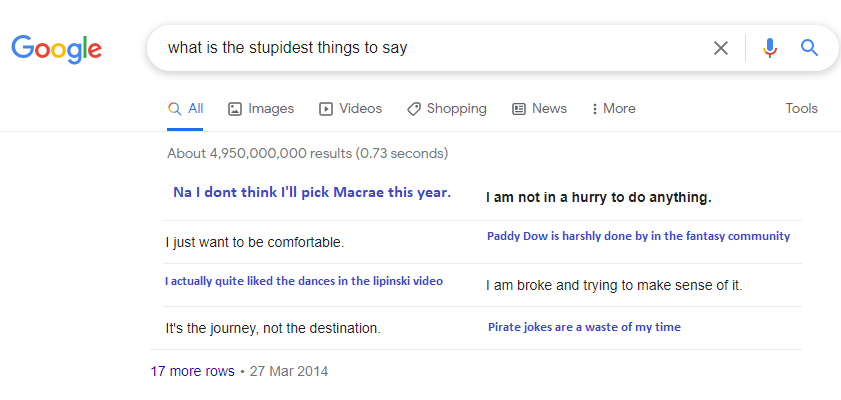This image depicts a Google search results page. The layout is in a landscape rectangular format without any borders, blending seamlessly into the white background. 

In the top left corner, the familiar multicolored Google logo is displayed, comprising blue, red, yellow, and green colors. To the right of the logo, the standard Google search bar is visible. It is a stretched oval or rectangular shape with curved edges, containing the search query, "what is the stupidest things to say?" This query is grammatically incorrect as it uses "things" instead of "thing." Next to the search bar on the right are the standard gray 'X' for clearing the search, the microphone icon with blue and red colors, and the blue search icon.

Below the search bar are the usual navigation tabs for Google searches. From left to right, these tabs read: "All," "Images," "Videos," "Shopping," "News," and "More," with "More" having three dots next to it. Another tab labeled "Tools" is positioned at the far right. The "All" tab is currently selected, indicated by the thick blue line beneath it and its blue text, while the other tabs and their respective icons are gray.

Directly under these tabs, a thin gray line spans the screen. Below this line, it states that there are approximately 4,950,000,000 results found in 0.73 seconds. The first result is a series of textual phrases divided into two columns.

In the left column:
1. "I don't think I'll pick McRae this year."
2. "Nah, I don't think so..."
3. "I just want to be comfortable."
4. "I actually quite like the dances in the Lipinski video." (in smaller blue text)
5. "It's the journey, not the destination."

In the right column:
1. "I am not in a hurry to do anything."
2. "Patty Dow is harshly done in by the fantasy community." (in smaller blue text)
3. "I am broken trying to make sense of it."
4. "Pirate jokes are a waste of time." (in smaller blue text)

Below these rows of text, left-aligned in blue font, it states "17 more rows" next to a gray dot, followed by the date "27 MAR 2014," suggesting a way to access more search results from that particular date.

The overall image gives a detailed view of a Google search results page, highlighting the layout, colors, and specific textual content displayed in the search results.